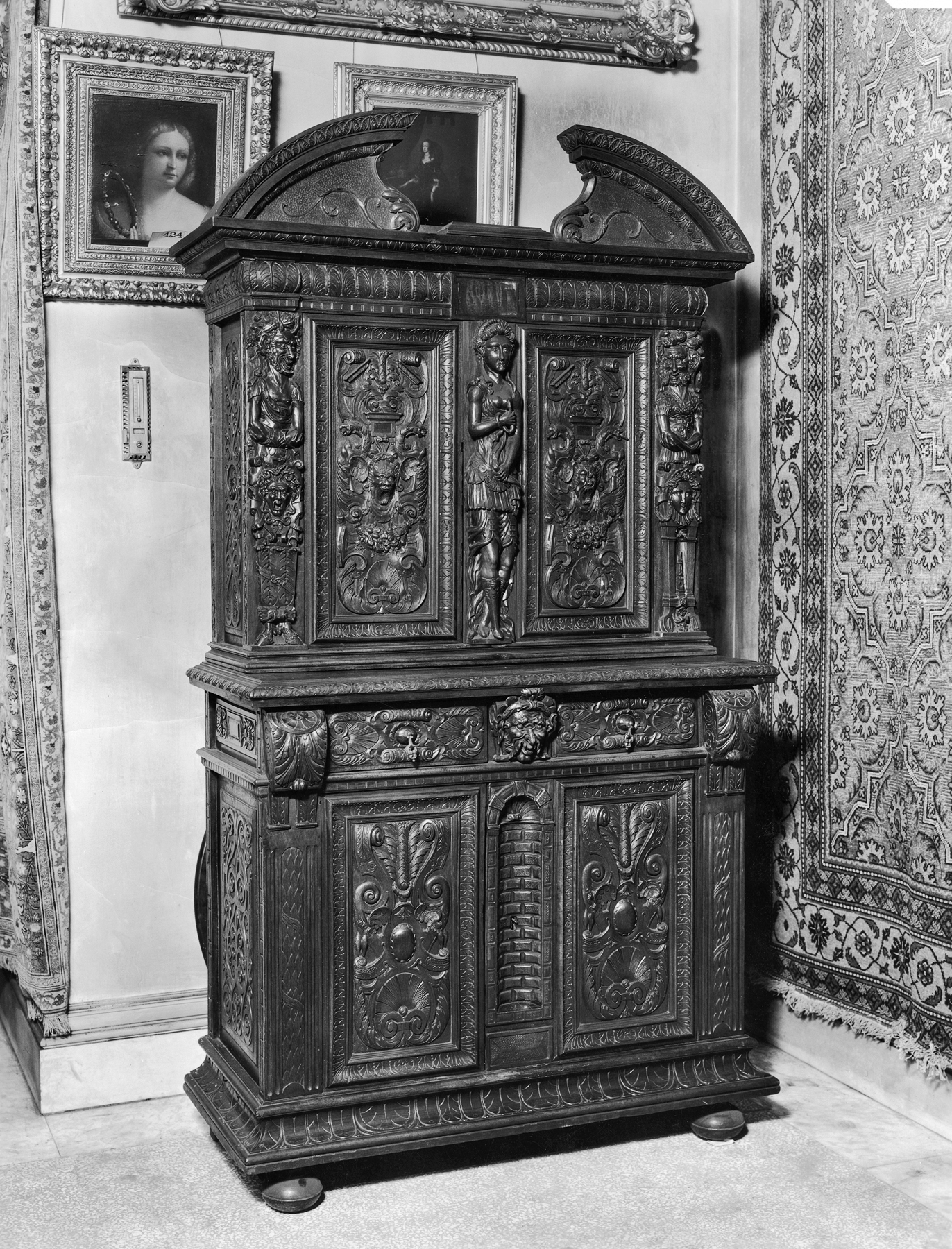This vintage black and white photograph captures a large, ornate piece of furniture, likely from the Victorian era, exuding a gritty, aged charm. The furniture, potentially made of metal or bronze, features an intricate and elaborate design. It is a two-tiered structure, with the bottom tier adorned with detailed plaques and a sculpted human head at the center. The top tier also carries plaques and is graced with three statues: a woman in the middle and two male or soldier figures on either side. Floral designs are etched both between the human sculptures and on the bottom tier. Despite its heavy and ornate appearance, the furniture does not seem to have any discernible drawers or openings, adding to its mysterious allure. The backdrop includes a detailed brick design and an ornately patterned rug on the wall to the left. Flanking the furniture on the wall are two framed photographs of women - one a close-up of a woman's head and chest, and the other a full-body portrait. The meticulous craftsmanship and rich decorative elements make this piece a fascinating relic from a bygone era.